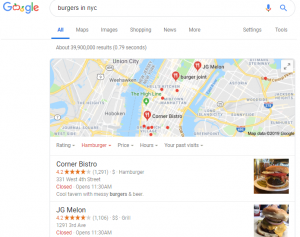The image is a screenshot of a Google search results page for "burgers in NYC, New York City." The Google Doodle of the day is creatively modified, with the first 'O' depicted as a red apple adorned with green leaves, and the second 'O' stylized to resemble a yellow fruit, perhaps a yellow apple, as it also features green leaves.

Below the search bar, the navigation tabs are highlighted: 'All' is lit up in blue, accompanied by 'Maps,' 'Images,' 'Shopping,' 'News,' and 'More.' To the right of these tabs, options for 'Settings' and 'Tools' are available for further customization.

In the main search results section, a map of New York City is displayed, prominently featuring the Hudson River and various boroughs. The map includes three pinpointed locations for popular burger restaurants. The first location, Corner Bistro, has a rating of 4.2 stars based on 1,291 reviews. Although it is currently closed, it is scheduled to open at 11:30 a.m. The second location, J.G. Melon, also boasts a 4.2-star rating and is similarly closed, with an opening time of 11:30 a.m.